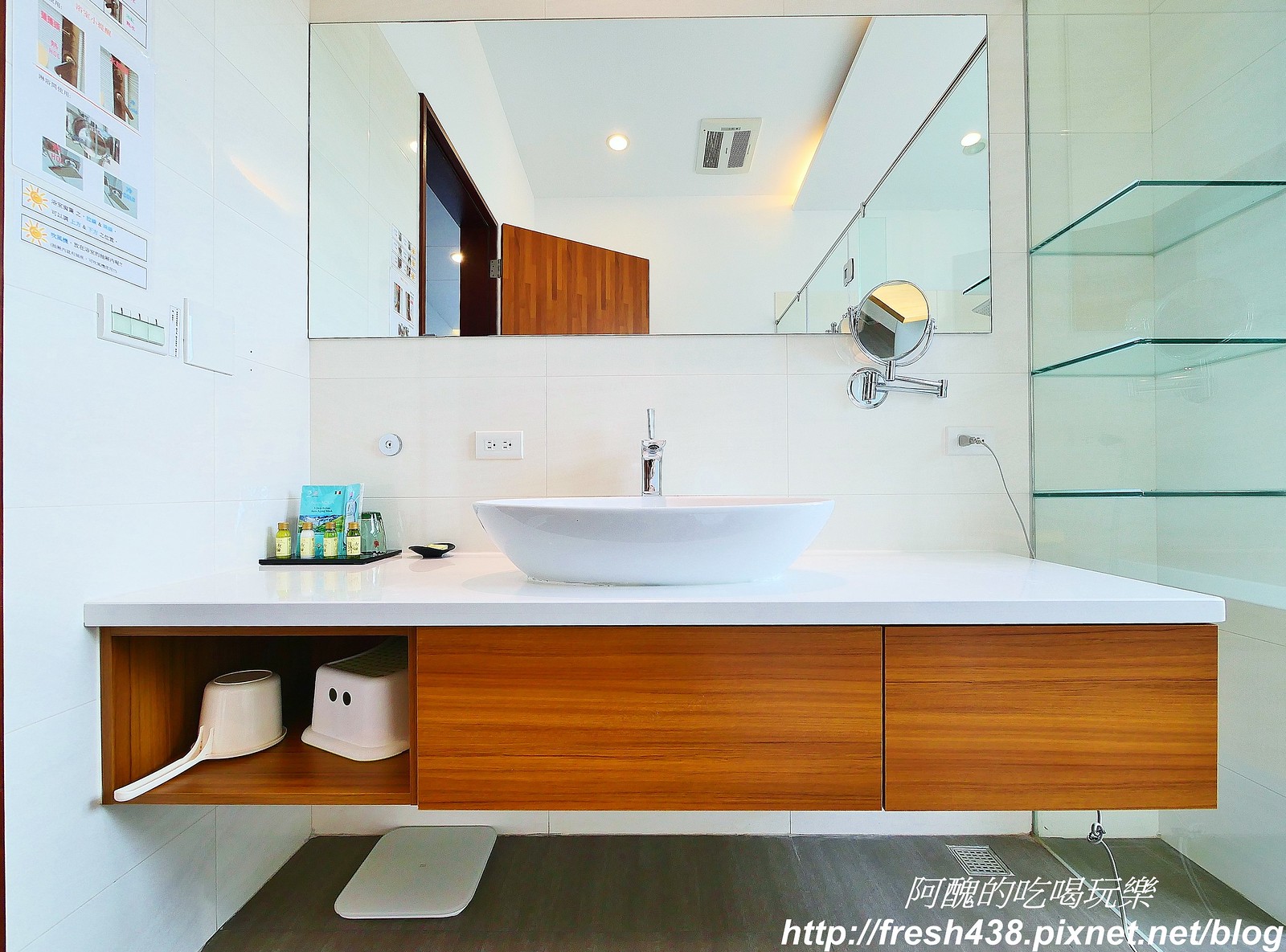The photograph depicts the interior of a bathroom, with the primary focus on a well-appointed sink area. The sink itself features a large, pristine white ceramic basin with a single nozzle faucet, perched elegantly atop a cultured marble countertop of matching whiteness. Behind the sink, a white tile backsplash stands tall at approximately six feet, extending all the way up the wall. Mounted on this backsplash is a substantial mirror, roughly four feet by three feet in dimensions, which reflects the rest of the bathroom. Below this main mirror, a smaller magnifying facial mirror is affixed to the wall, offering a convenient grooming aid.

In the right section of the image, a series of three glass shelves are visible, supported by sleek silver poles, providing storage space for bathroom essentials. The base cabinetry of the sink is crafted from a pine-colored wood, adding a warm natural contrast to the predominantly white décor. An open section on the left side of the cabinet reveals a couple of plastic devices, hinting at stored toiletries or cleaning supplies. The overall arrangement of elements and choice of materials in this bathroom demonstrates a blend of functionality and aesthetic appeal.